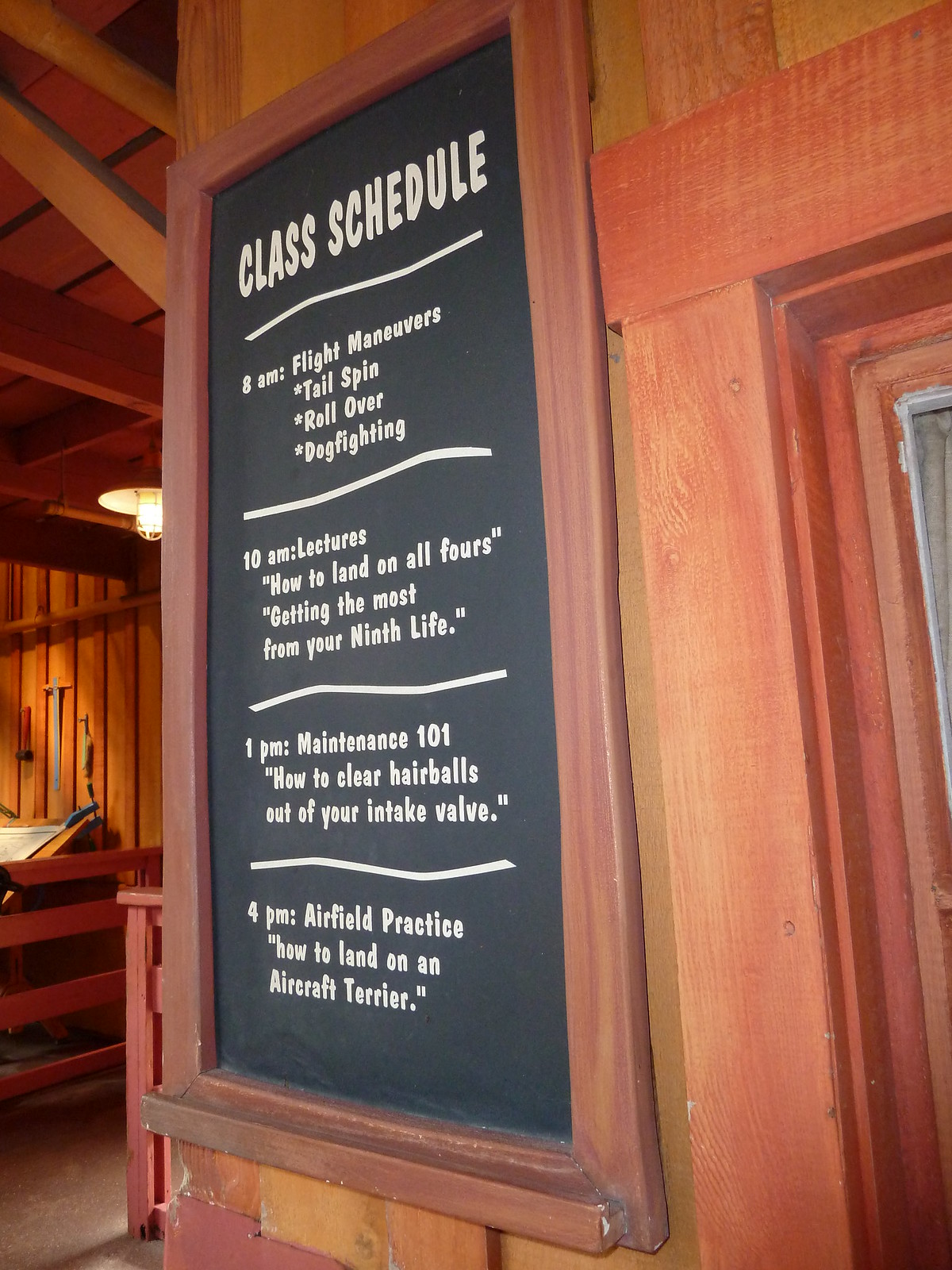The photo captures an indoor setting within what appears to be a log cabin decorated predominantly with cherry-colored wood. The central focus is a photographic sign, printed and mounted on a blackboard, which is affixed to a wooden wall. This wall, adjacent to a wooden-framed doorway, provides a glimpse into another room featuring a fence-like structure and buildings. Above the entrance, under an electric light hanging from a ceiling lined with wooden rafters, the blackboard displays a catchy class schedule written in white text. The schedule lists:

- **8am**: Flight Maneuvers - "Tailspin," "Rollover," and "Dogfighting"
- **10am**: Lectures - "How to Land on All Fours" and "Getting the Most from Your 9th Life"
- **1pm**: Maintenance 101 - "How to Clear Hairballs Out of Your Intake Valve"
- **4pm**: Airfield Practice - "How to Land on an Aircraft Terrier"

The setting inside the cabin is cozy and multifunctional, with visible colors including white, black, brown, tan, and yellow, suggesting diverse uses and a touch of whimsy as indicated by the whimsical schedule.